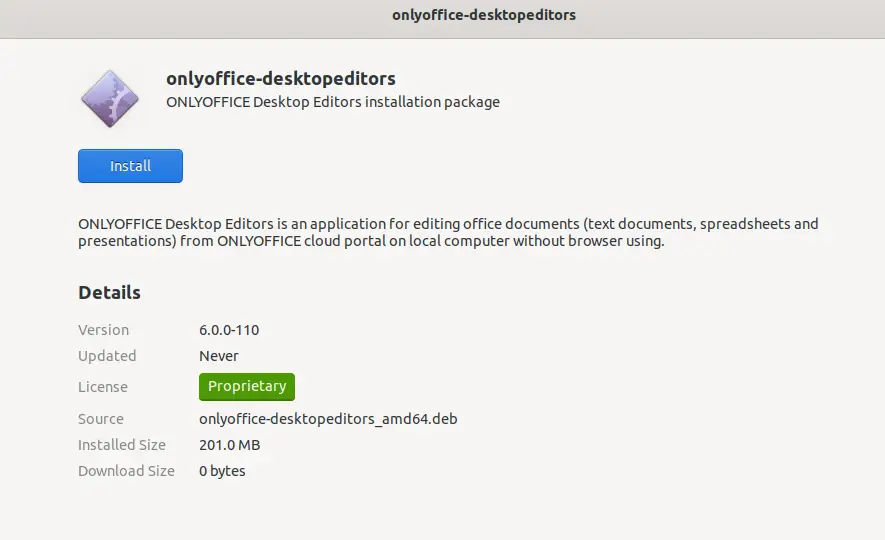The webpage displayed is dedicated to OnlyOffice Desktop Editors, showcasing an application for editing office documents, spreadsheets, and presentations locally without a browser. At the very top, a gray bar spans the width of the page, prominently displaying "OnlyOffice Desktop Editors." Below this bar, in the upper left corner, the phrase "OnlyOffice Desktop Editors" reappears alongside a square logo featuring a pink background with small gear icons.

Beneath these headings, the page reads "OnlyOffice Desktop Editors Installation Package." Adjacent to this description on the left side is a blue install button.

The detailed description reads: "OnlyOffice Desktop Editors is an application for editing office documents, text documents, spreadsheets, and presentations from OnlyOffice Cloud Portal on a local computer without using a browser."

Further app details include:
- Version: 600-110
- Updated: Never
- License: Proprietary (highlighted in a green square)
- Source: OnlyOffice_Desktop_Editors_AMD64.DEB
- Installation Size: 201.0 megabytes
- Download Size: 0 bytes

The .DEB file indicates that this installation package is intended for Linux or Ubuntu systems.